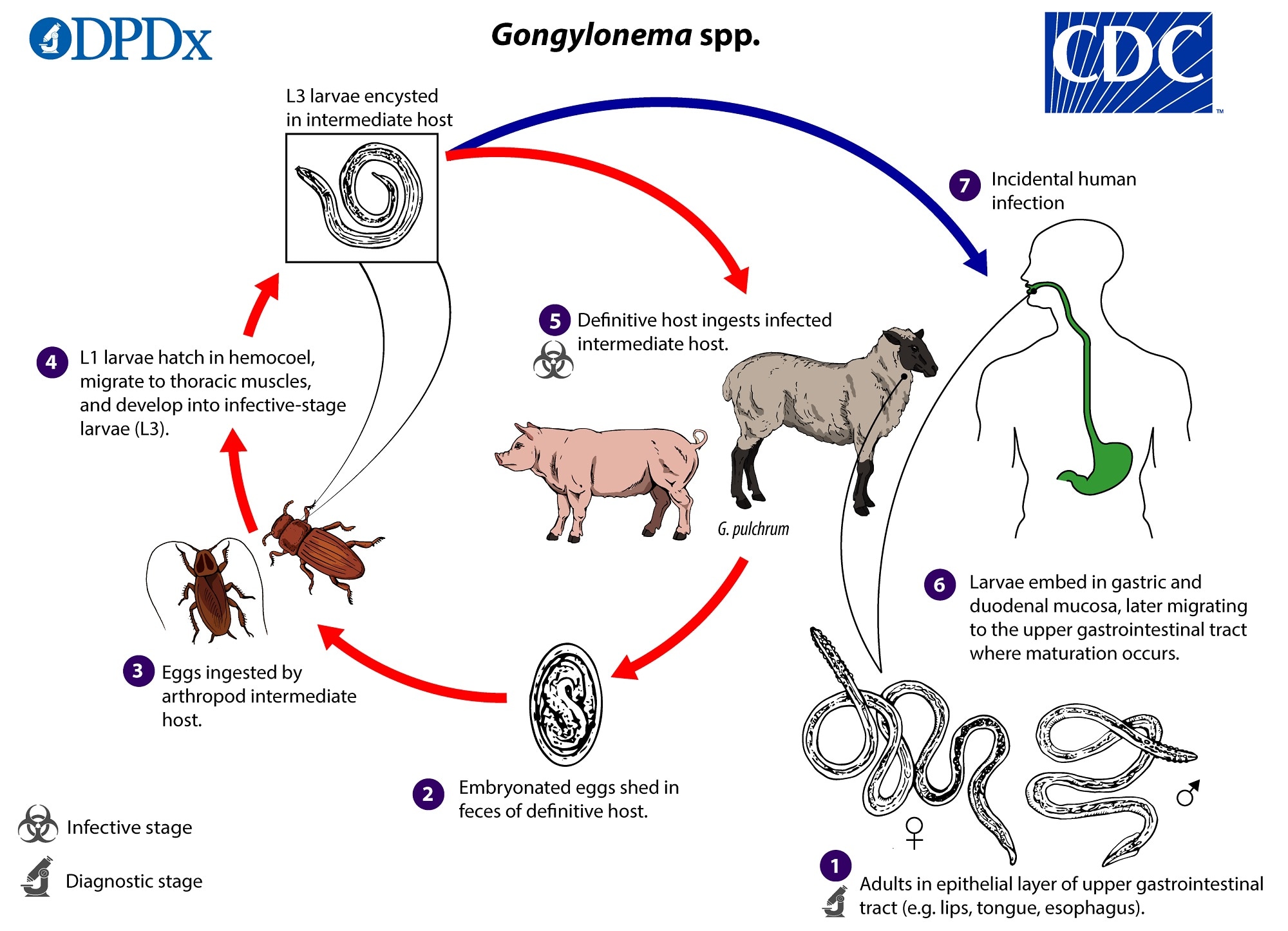This detailed chart, produced by the CDC and labeled with its logo in the upper right corner and a "DPDx" microscope icon in the upper left, illustrates the life cycle of the parasite Gongylonema spp. Starting from the top, the cycle begins with the adult worm residing in the upper gastrointestinal tract of a host, which can be an animal such as a pig or sheep, or a human. Eggs from the adult worms are shed in the host's feces, depicted by red arrows leading to their ingestion by intermediary hosts, such as cockroaches or other arthropods. Within these arthropods, the eggs hatch into larvae. Another set of red arrows shows these intermediate hosts being subsequently consumed by larger mammals, including pigs, sheep, and potentially humans. The larvae then embed themselves in the gastric and duodenal mucosa of these new hosts, migrating to the upper gastrointestinal tract where they mature into adult worms, thus completing the cycle. The chart also distinctly labels various stages as either "infective" or "diagnostic," providing a comprehensive overview of the parasite's life cycle and transmission pathways.